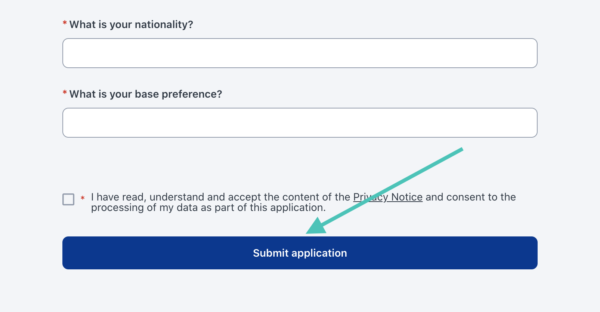This image displays a form page designed for user input within a digital application setting. The photograph is portrait-oriented and features a gray background devoid of borderlines. 

At the top of the form, a mandatory question in black text reads, "What is your nationality?" followed by a red asterisk indicating its required status. Directly below, there is a long, rectangular text box with a gray border and rounded edges intended for user input.

The next mandatory question, also marked with a red asterisk, asks, "What is your base preference?" It is followed by an identical text box for entering a response.

Beneath this is a gray checkbox with an accompanying asterisked statement: "I have read and understand and accept the content of the privacy notice and consent to the processing of my data as part of the application." This indicates a necessary agreement for proceeding.

At the bottom of the form is a blue rectangular button with rounded edges, featuring white text that reads "Submit Application." Positioned just above this button is a green arrow pointing downwards towards the "Submit Application" text. This arrow originates beneath the second text box on the right side and angles downward to the bottom left, visually guiding users to the submit button to continue to the subsequent page.